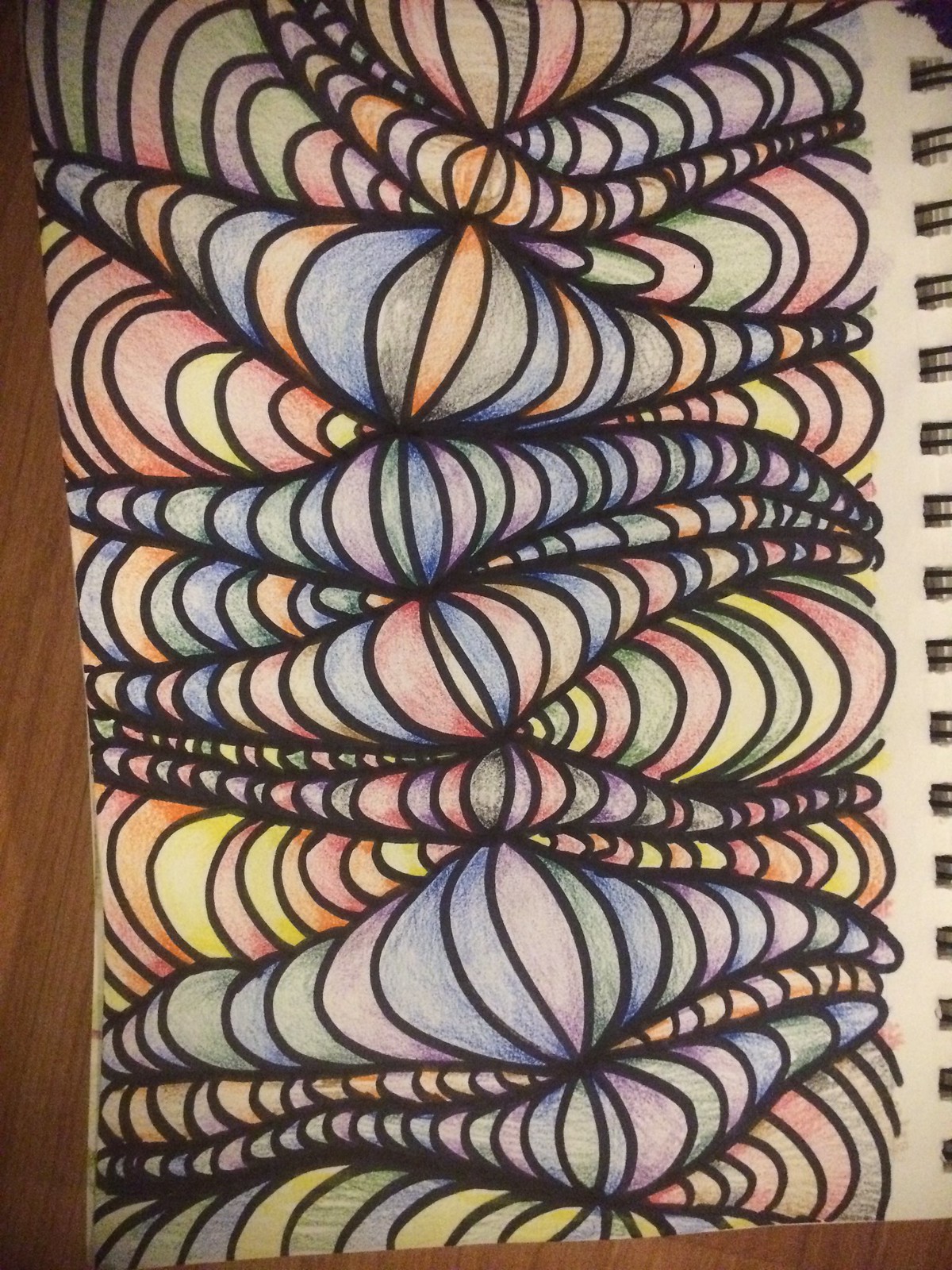This photograph showcases a vertical-rectangular page from a sketchbook resting on a medium brown wooden table. The spiral binding is visible on the right, indicating the sketchbook is positioned backwards. The design on the white page is modern and portrays a dynamic array of three-dimensional, interwoven circles and spirals. These shapes start narrow on the sides and gradually broaden toward the center, creating a wave-like pattern that gives a sense of depth. The circles, intricately drawn with pencils, display a vibrant palette including light blue, gray, orange, green, yellow, light green, dark green, pink, and red. The colors create a layered effect where light shades appear closer to the viewer, while darker ones recede, adding to the three-dimensional appearance of the sketch. The composition is devoid of text, focusing purely on the detailed and colorful abstract designs.